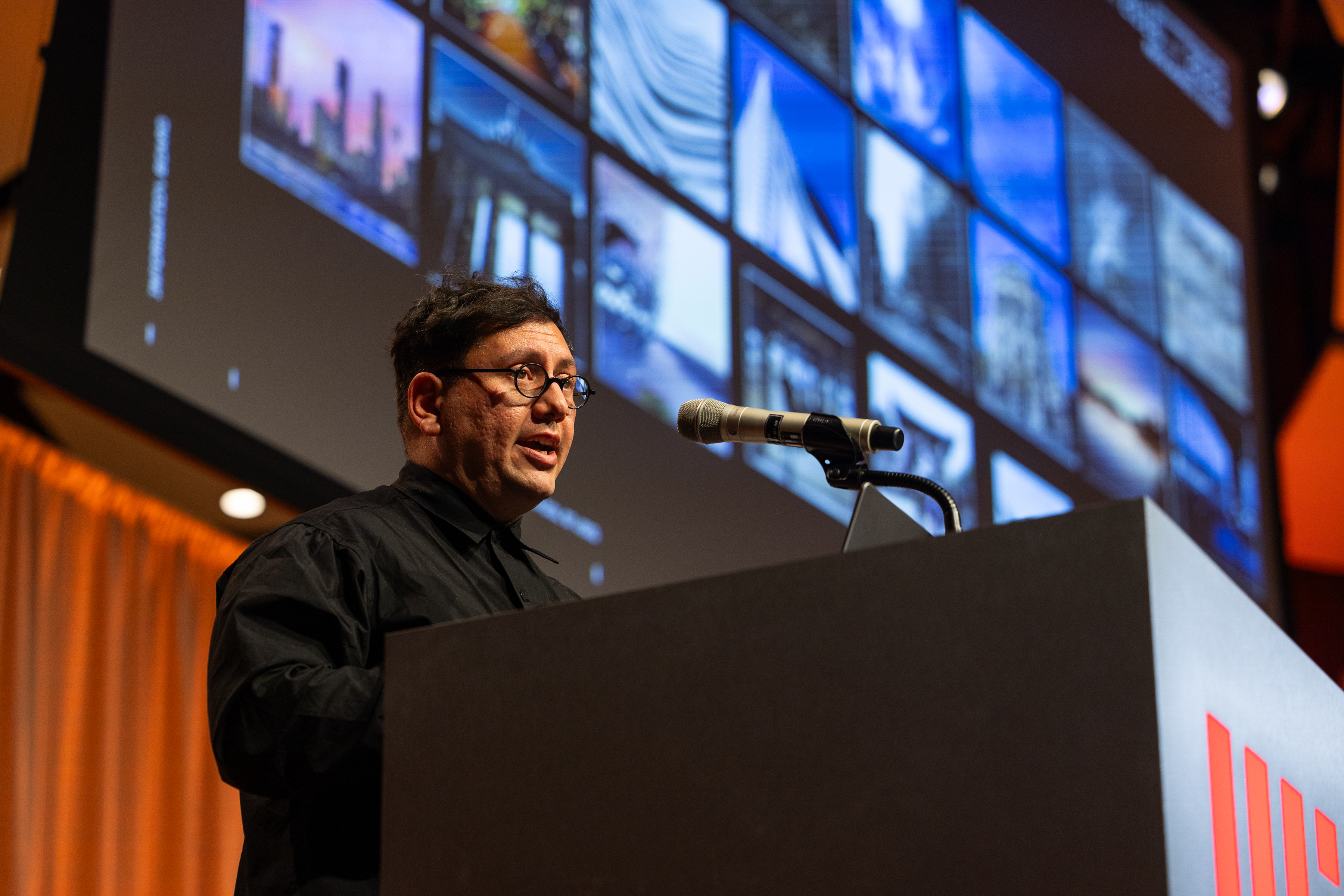This horizontal photograph captures an image of a man, possibly in his late 40s and of Hispanic or Indian descent, delivering a speech at a podium. The photo is taken from a side angle, slightly upward, emphasizing the speaker and his presence. The podium's side is brown, while the front is dark gray with blocky letters that potentially spell out "MIT" in orange print in the lower right corner. The man, who has short black hair, small circular-rimmed glasses, and is wearing a black, fully buttoned shirt, has his mouth open as if mid-sentence. A silver microphone on a black rod extends towards him from the top of the podium. Behind him, a large rectangular screen with three rows of square images, likely architectural, is mounted on the wall, and an orange curtain underneath adds a contrasting color to the scene. The screen shows a variety of images, including city buildings and curved lines, contributing to the setting's academic or professional ambiance.